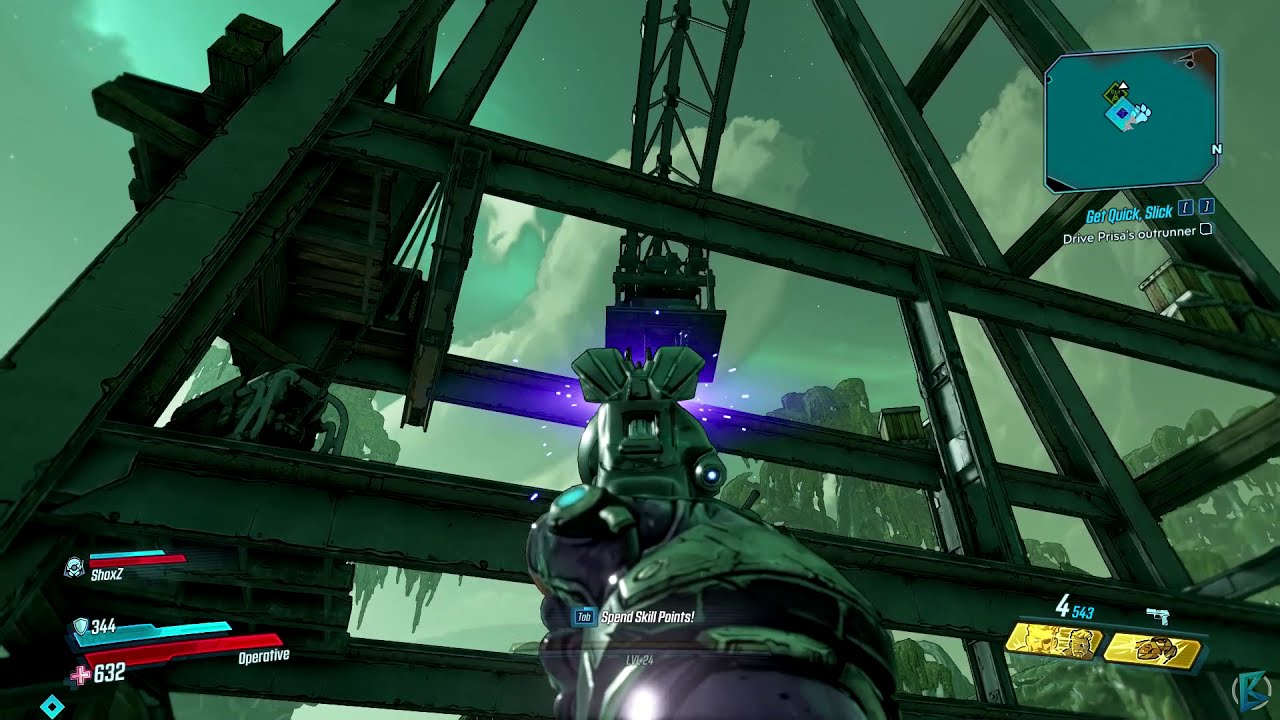The image is a detailed screenshot from a shooter video game, showcasing its vibrant and complex interface. Central to the bottom of the screen, a robot with a green body, grey bottom, and prominent ears faces away from the viewer, staring towards a towering metallic frame and crane extending from the top down to the center of the image. The sky above is a mix of blue and bluish-green hues, dotted with white clouds. In the foreground, a hand is wielding a pistol either having shot or about to shoot at the tall metallic structure, causing a striking violet explosion. The game's HUD (heads-up display) is rich with information: in the bottom right corner, a gun symbol appears with the number four; the bottom left corner displays lines colored turquoise and red, showing stats like a turquoise line at 344 and a red line, likely representing health, at 632. Additionally, labels such as "Shaq C632-344 operative" are visible. The upper right contains more game data, with terms like "get quick sick" and a turquoise square, complemented by two red squares in the lower right. The background, aside from the industrial structure, includes tree silhouettes in various shades of green, enhancing the immersive, industrial environment.